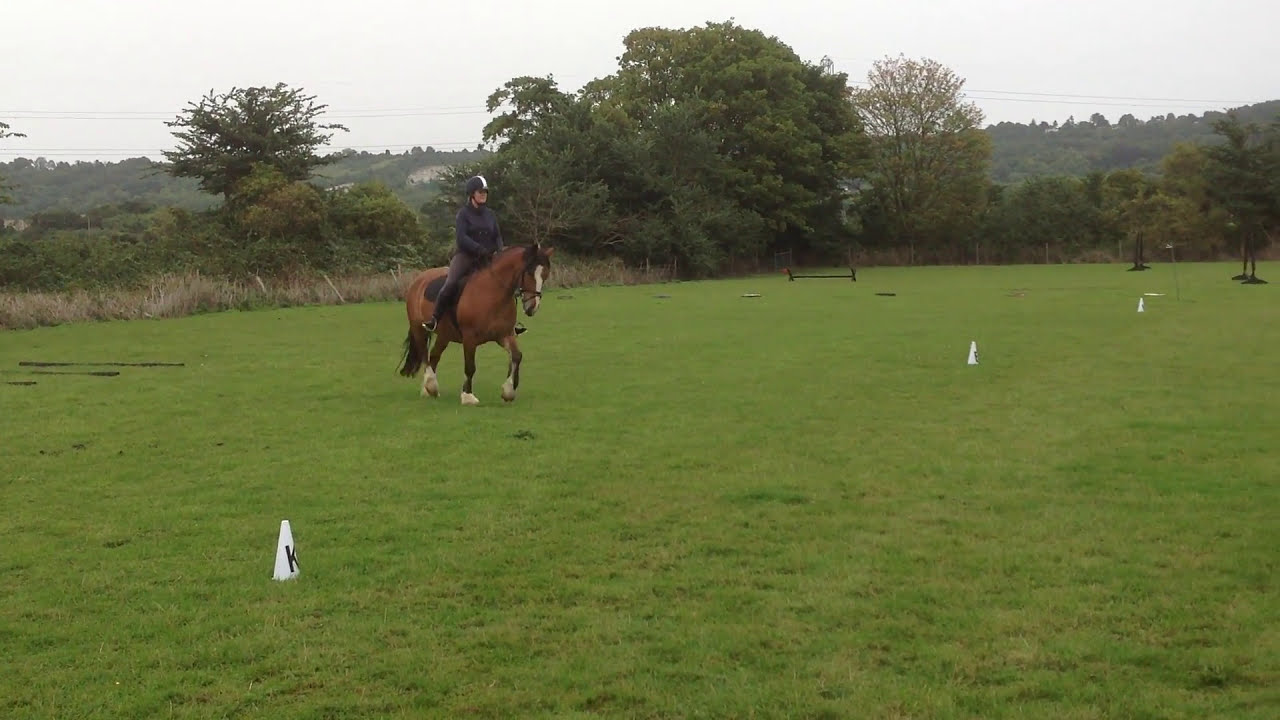A vibrant, full-color outdoor photograph captures a lively equestrian event set on a lush, expansive green grassy field. In the middle of the field stands a robust brown horse adorned with distinctive white spots on its muzzle and the lower parts of its legs. Seated atop the horse is a rider, dressed in a full black ensemble including slacks, shoes, and a jacket, complemented by a black helmet with a white stripe running up the middle. Scattered across the vivid green grass are several small white cones with black letters, such as K and B, which mark positions in the field. Just beyond the borders of the field are dense, lush trees with green, fluffy leaves, contributing to the serene backdrop. The sky above is mostly clear and light blue, although some descriptions suggest it might be somewhat hazy or overcast, adding depth to the atmosphere of the photograph. Overall, this image vividly documents an engaging moment in an equestrian setting, surrounded by nature's verdant beauty.